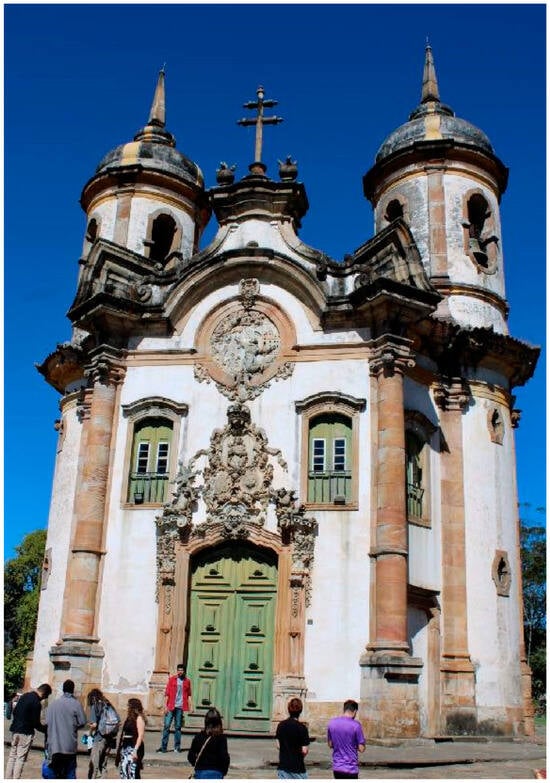This photograph, taken in portrait mode, captures the exterior of an old church, likely dating back to the 15th or 16th century. The church features a smooth white stone front façade accented with tan, brown, and black elements. Its architecture includes two cylindrical steeples capped with pointed towers and round domes, likely bell towers, adorned with small windows and turrets. A stylized double cross is prominently situated at the center above the entrance. The entrance itself showcases a green, elaborately arched door with matching arched window recesses. The background reveals a clear blue sky and some trees, enhancing the historical and serene ambiance. In front of the church, a group of nine people is gathered. Seven of them are lined up, collectively viewing the church, while another stands near the green door, facing away from the building. This individual is distinct in their red shirt and blue jeans. Among the group, another person stands out in a bright purple t-shirt, while the others are dressed in gray or black shirts. This detailed scene encapsulates both the architectural grandeur of the church and the diverse group of onlookers.